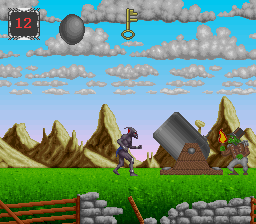This square artwork features a dynamic scene set against a red-hued background. In the top left corner, the number "12" is prominently displayed in black. Dominating the center of the composition is a gray creature, oriented to the right. On the left side of the image, a dramatic canyon is depicted, its gray walls contrasting with the adjacent brown terrain. To the right of the canyon, a character clad in green is depicted wearing brown armor. This character is raising a red torch with its right hand, adding an element of mystery and action to the artwork.